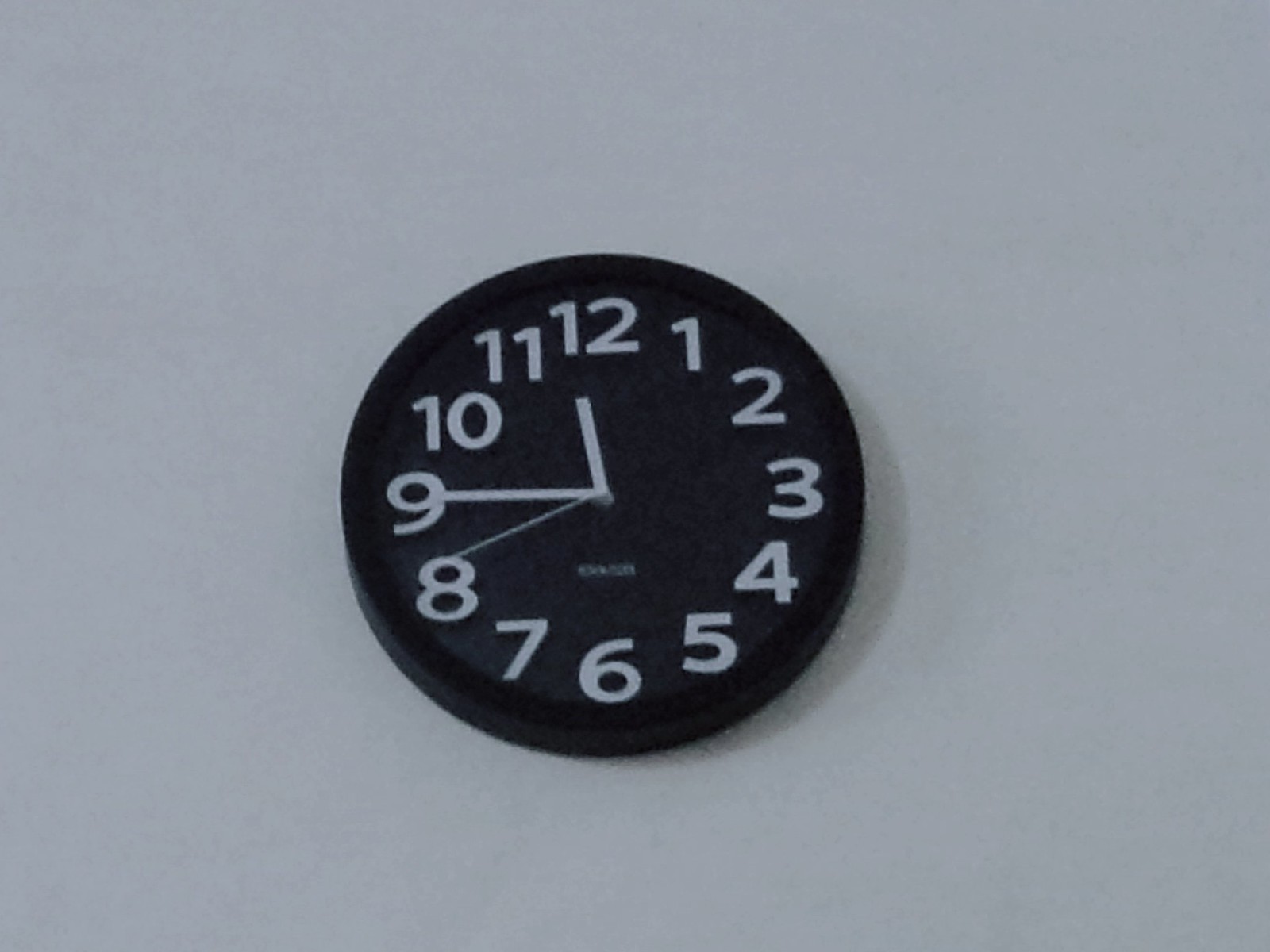This image features a black, analog clock mounted on a white wall. The clock prominently displays large, white numbers from 1 to 12, making it easily readable from a distance. The clock hands are also white, with the larger hand pointing at the 9, the smaller hand positioned between 11 and 12, closer to 12, indicating the time is 11:45. The second hand is slightly past the 8, marking the 40-second point. There's a small, indistinguishable text right above the 6. The clock appears slightly angled, casting a subtle shadow on the right side, emphasizing its three-dimensional presence against the plain background.